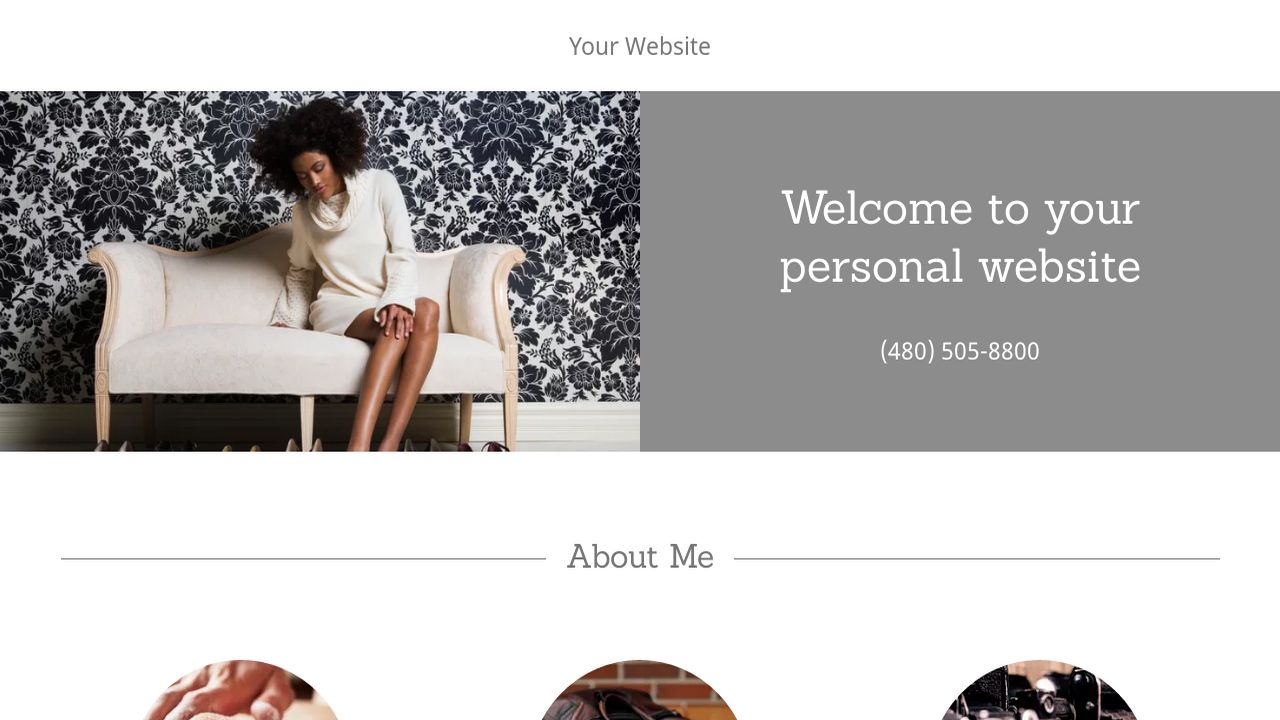The image showcases a website template designed for personal web pages. At the very top, the header, written in a subdued gray font, reads "Your Website." The header itself is split into two distinct sections. On the right side, set against a gray background with white font, the text warmly greets visitors with "Welcome to your personal website." Below this greeting, a contact phone number is prominently displayed: 408-505-8800.

On the left side of the header, a striking photograph captures attention. It features a slender Black woman, likely a model, with a natural hairstyle consisting of an impressive, large afro. She is elegantly attired in a white mini dress with a cowl neck and long sleeves, seated on a light beige Victorian-style upholstered sofa. The background hints at an ornate setting, with vivid, large, and small gray flowers patterned on the wallpaper.

Directly below the header, against a white background, the centered text reads "About Me," flanked by thin horizontal lines on either side. The content beneath this point is partially visible, hinting at additional sections. Three circular images peek from the bottom edge of the visible area, with the middle one showing two rows of red bricks against mortar. The other two images are too obscured to identify further.